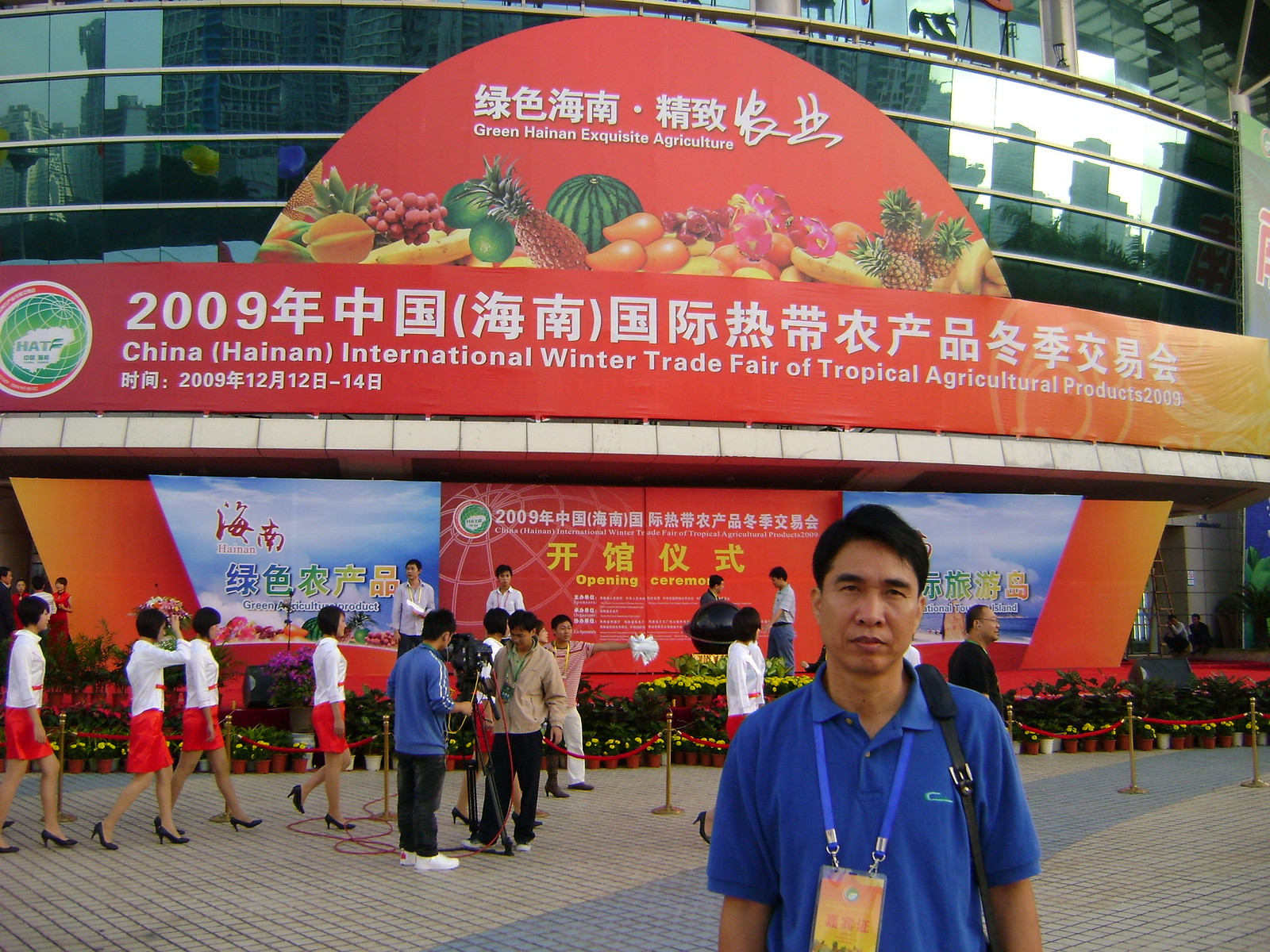In the photograph, an Asian-looking man stands in the foreground, appearing slightly unenthused, with his eyes squinting towards the camera. He has dark black hair parted from left to right, dark brown skin, and dark eyebrows. He is dressed in a short-sleeved blue shirt with a collar, adorned with a blue lanyard from which a yellow and orange card hangs. Over one shoulder, he carries a strap with a silver buckle. The lower part of his hand is cut off at the bottom of the image. The ground beneath him is covered in a mosaic of closely packed tiny tiles, primarily gray, with a line of blue ones.

Behind him, a rope barrier on metal posts lines up a group of women who appear to be in uniform, dressed in white shirts, red skirts, and black heels, possibly flight attendants. Nearby, a man in a blue shirt, black pants, and white shoes adjusts his camera equipment, while another man stands to the left, donning a gray coat, light brown long-sleeved shirt, and blue pants.

The backdrop features a large, architecturally striking building with a prominently curved, glass-covered façade divided by three sections of siding. At the top of the building, a grand banner transitions from red on the left to yellow on the right, resembling the outline of an orange. The banner reads "2009 China Hainan International Winter Trade Fair of Tropical Agricultural Products 2009," accompanied by Chinese characters and the phrase "Green Hainan, Exquisite Agriculture." Above this text is a half-circle design showcasing an array of fruits and vegetables.

Several people milling about suggest the buzz of an ongoing event, lines forming to enter beneath the banner. There is a stage visible behind the main figure, with signage possibly indicating an opening ceremony.